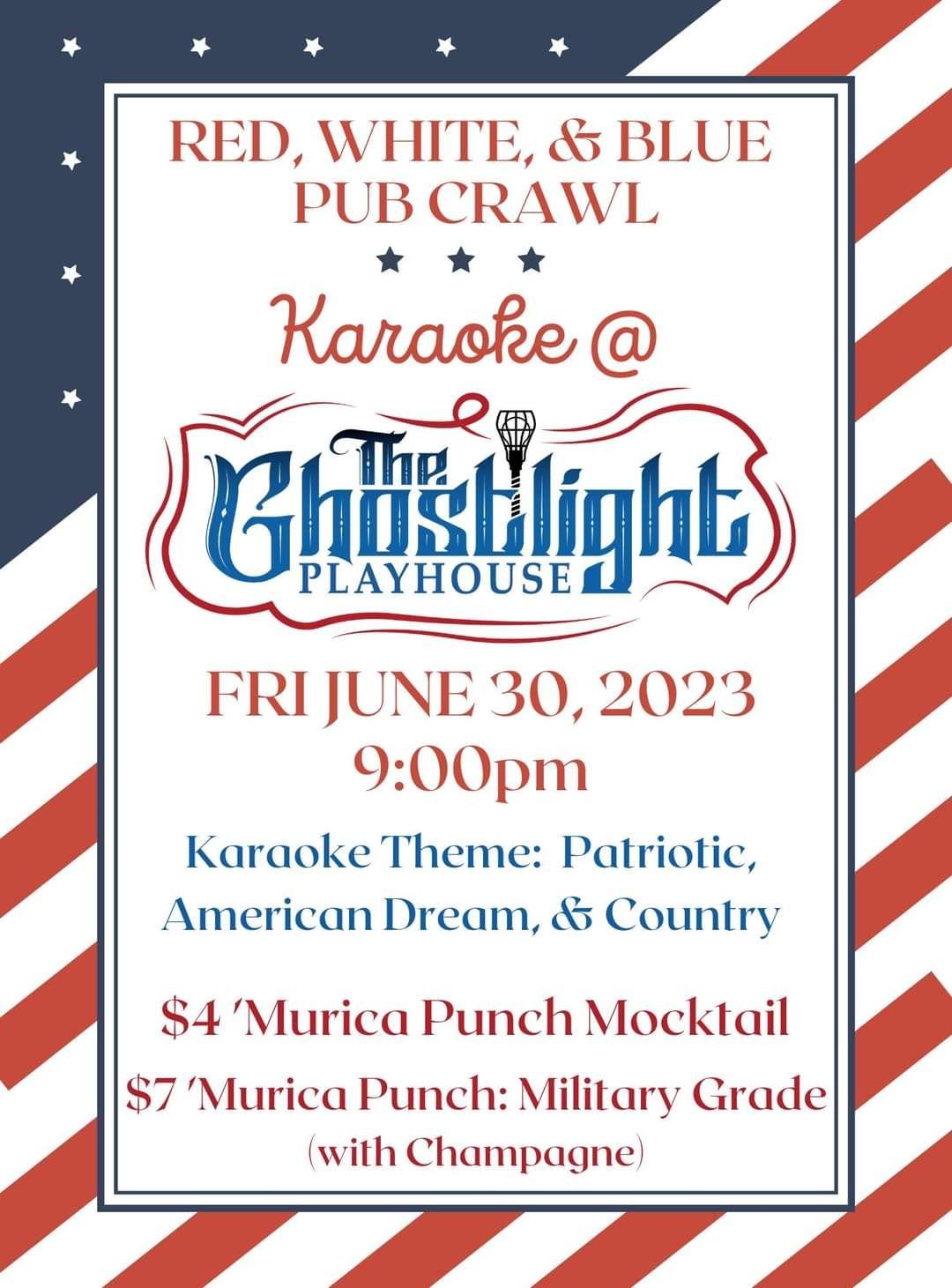This vibrant poster designed in the style of the American flag features a triangular blue field with white stars in the top left corner, and diagonal red and white stripes running from left to right. At the center of this patriotic background lies a bordered white area containing detailed event information. The top of this central section has bold red text that reads "Red White and Blue Pub Crawl" above three black stars. Below, in elegant cursive, the text announces "Karaoke at," followed by "The Ghost Light Playhouse" in a red-bordered image in blue writing. Further down, it states in red lettering, "Friday, June 30, 2023 at 9 PM," with the following blue text detailing the karaoke themes: "Patriotic, American Dream, & Country." The poster also advertises drink specials, noting in red type "$4 Mauritia Punch Mocktail" and "$7 Mauritia Military Grade Punch with Champagne." This eye-catching poster effectively combines patriotic elements to promote an American-themed pub crawl and karaoke night.